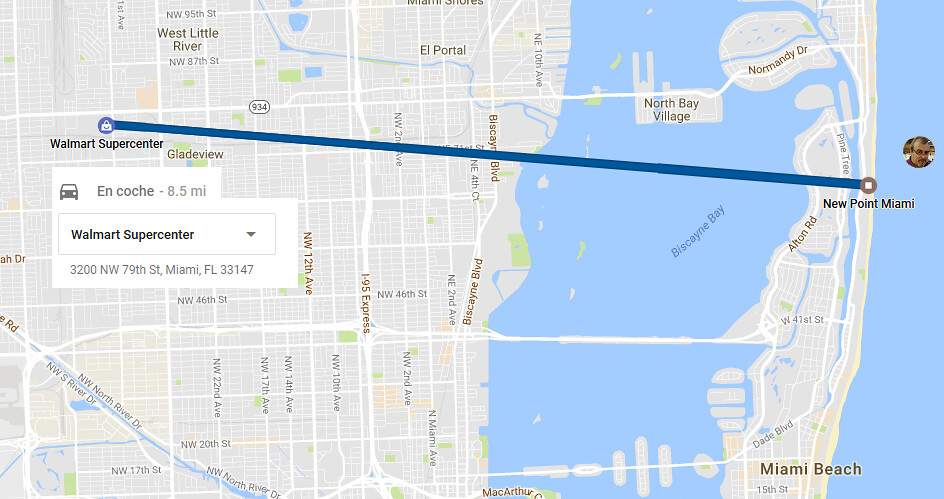The image depicts a detailed map highlighting the route to a Walmart Supercenter. Starting from the left, the path traverses halfway across the map, then descends from the top, veers slightly left, and continues downwards to the bottom left quadrant of the map, just left of the center. The map features a large landmass shaded in light white, with numerous white lines representing streets and thicker white lines indicating the Expressway.

Approximately a third of the map on the right side is colored light blue, symbolizing water. Near the top right corner, there is a small pin about two inches from the top, which features a man's face with glasses and dark hair. Below and to the left of this pin, there's a brown circle with a white square inside it, labeled "New Point Miami."

From "New Point Miami," a thick deep blue line extends leftward, nearly spanning the width of the map. The Walmart Supercenter is marked along this blue line, situated about a third of the way down. Adjacent to the blue line is an island named "North Bay Village," and further up and to the right, another island named "Normandy Drive" is marked, lying close to the landmass on the right side of the map.

The visual elements, including detailed roads, landmarks, and water bodies, all contribute to guiding someone to the Walmart Supercenter effectively.